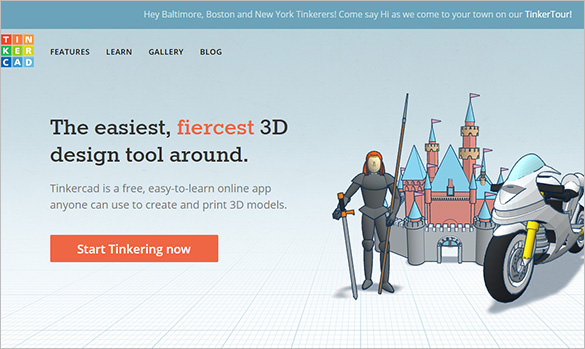The image displays a vibrant and inviting website interface for Tinkercad that is predominantly rectangular and horizontally oriented. 

At the top of the interface is a grayish-blue banner featuring the text: “Hey Baltimore, Boston, and New York tinkerers, come say hi as we come to your town on our tinker tour.” Below this banner, the background transitions from gray at the top to white towards the bottom.

In the top-left corner, there is a colorful logo composed of letter blocks which spell out "T-I-N-K-E-R” in a gradient of red, orange, green, yellow, and blue hues. Adjacent to the logo are black navigation links reading: “Features,” “Learn,” “Gallery,” and “Blog.”

In the center-left of the page, there is a prominent slogan in black text, “The Easiest, Fiercest 3D Design Tool Around,” with the word “Fiercest” highlighted in red. Below this slogan, in smaller black text, it is stated, “Tinkercad is a free easy to learn online app anyone can use to create and print 3D models.”

A vibrant orange rectangular button below the text invites users to “Start Tinkering Now.”

To the right side of the page, a digital art image features a knight adorned in body armor (with a red-haired head exposed) holding a sword pointing towards the ground in his right hand and a joust stick or javelin in his left. Behind the knight is a whimsical castle in shades of pink, gray, and light turquoise. To the far right of the castle, a modern-day white motorcycle with yellow shocks and black tires contrasts with the medieval scene.